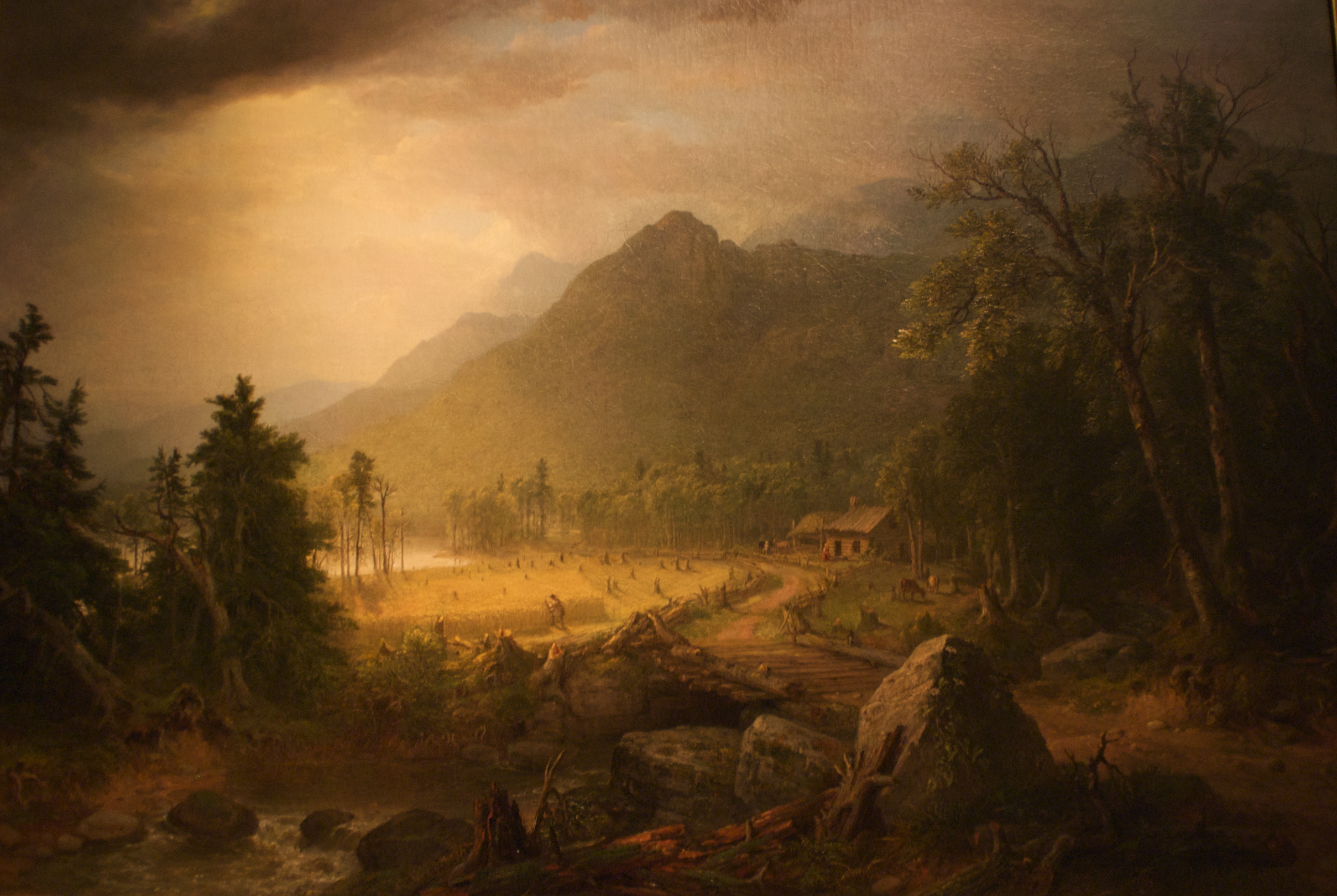The painting depicts a sprawling tropical village beach scene from an elevated vantage point, likely from a hill or rocky outcrop. In the foreground, large boulders, roughly the size of small cars, along with branches and tall grasses, frame the view. A rugged dirt road meanders down the hill, leading the eye towards a wide sandy beach bustling with approximately 25 indistinct human figures engaged in various activities. A rustic wooden bridge crosses a small stream connecting to the path, which then winds through a heavily forested area towards the shore.

On the right side of the scene, a small hut with a triangular roof equipped with a chimney and two windows faces the beach. Nearby, there appear to be some animals close to the hut, adding to the village atmosphere. Trees densely populate both sides of the painting, stretching right up to the beach edge. In the background, majestic mountains, perhaps volcanic in origin, reach their peak, partially covered in earthy tones and lush greenery, providing a dramatic backdrop. The overall image is rendered in a warm, sepia hue, adding an aged, nostalgic charm to the tropical tableau.